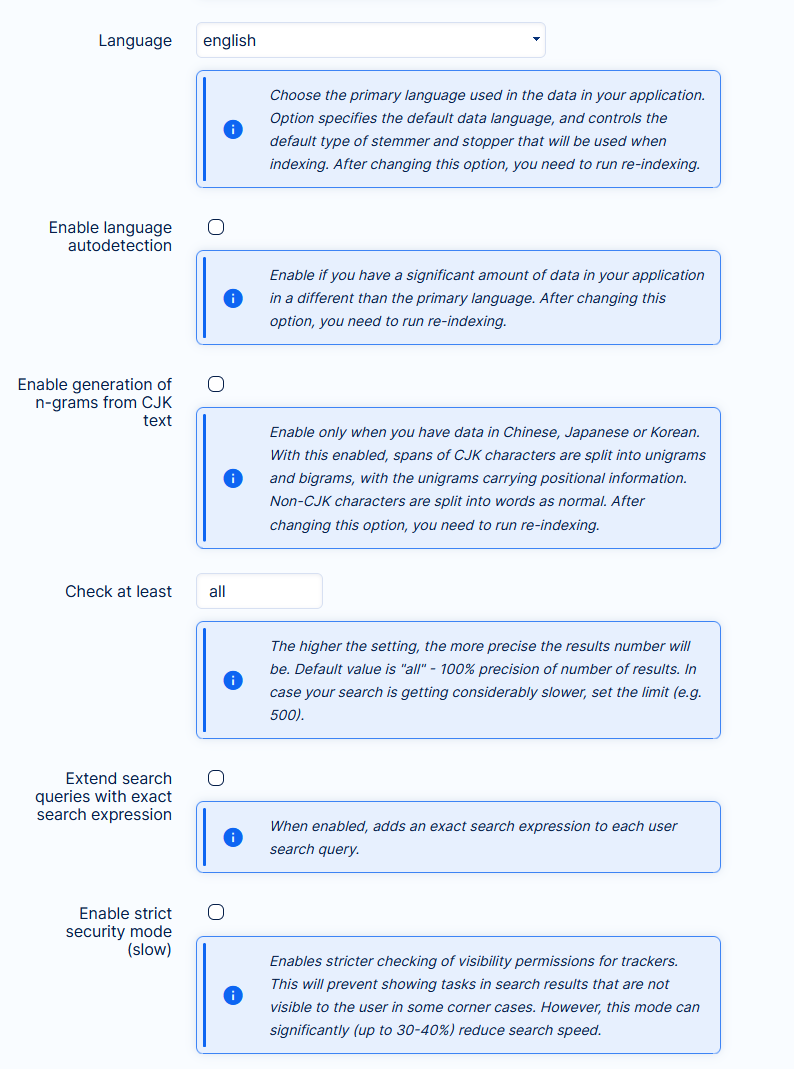At the top of the interface, there is a white drop-down menu labeled "english" (with a lowercase 'e'). To the left, in black lettering, it reads "Language." Beneath this, there's a rectangular area shaded light blue with a darker blue border and slightly rounded corners. 

On the left side, there is a bold blue line adjacent to a blue-filled circle containing a white 'i' for information. Next to this, in small italicized black font, the text reads: 

"Choose the primary language used in the data in your application. This option specifies the default data language and controls the default type of stemmer and stopper that will be used when indexing. After changing this option, you need to run re-indexing."

Below this information, there is an unselected radio button with the label "Enable Language Auto-Detection" in black text to the left. To the right, in a similarly styled light blue rectangular box, it states:

"Enable if you have a significant amount of data in your application in a different language than the primary language. After changing this option, you need to run re-indexing."

Further down, there is another unselected radio button next to a heading that reads "Enable Generation of N-grams from Capitalized CJK Text." Beneath this heading, there is another light blue rectangular area indicating:

"Enable only when you have data in Chinese, Japanese, or Korean. With this enabled, spans of capitalized CJK characters are split into unigrams and bigrams, with the unigrams carrying positional information. Non-capitalized CJK characters are split into words as normal. After changing this option, you need to run re-indexing."